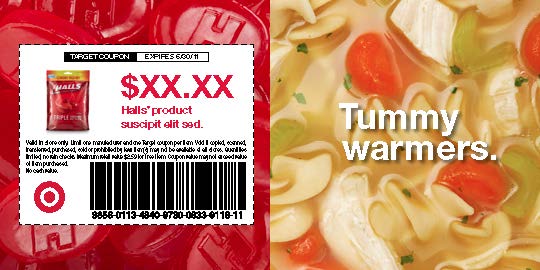This image features a bilingual promotional coupon for Halls Triple Action Cough Drops, prominently displayed in a split-screen layout. On the left side of the image, there's a striking backdrop of red Halls cough drops set against a white background. Central to this part, a coupon showcases a red bag of Halls Triple Action Cough Drops with text indicating a "Target coupon" which expires on June 30, 2011. The coupon includes a placeholder amount denoted as "XX.XX" off any Halls product. Additionally, a small Target icon is situated at the bottom left corner of the coupon, reinforcing the store association.

The right side of the image presents a close-up view of a bowl of chicken noodle soup, emphasizing the warmth and comfort it offers. Overlaying this cozy image is the phrase "Tummy Warmer," which connotes the soothing, stomach-settling qualities of the soup. This dual imagery adeptly aligns the relief provided by Halls cough drops with the comforting effects of chicken noodle soup, subtly suggesting a holistic approach to alleviating cold symptoms.